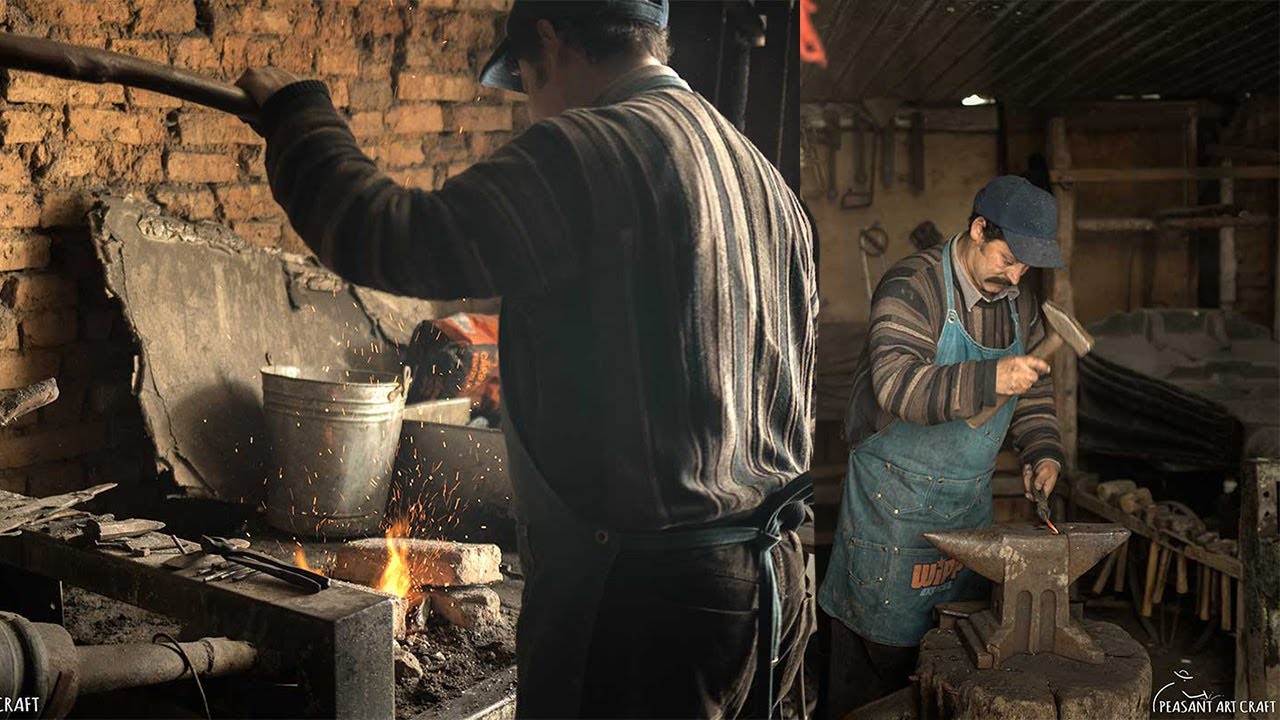In the digitally-created image of a small workshop, two men, who appear to be blacksmiths, are diligently working. The man to the left is tending to a charcoal fire, using a bellow to intensify the heat. He is partially obscured, with his back turned to the viewer, showing a striped shirt, blue jeans, a leather apron, and a blue baseball cap. A couple of bricks and a tin bucket are positioned next to him, amid various tools and structures indicative of an old, well-used foundry.

To the right, another man is focused on hammering a piece of metal on an anvil. He is adorned in a simple, round-striped sweater, a heavy blue apron, and a matching blue baseball cap, revealing dark hair and a mustache. The scene is set against a backdrop of aged red brick walls, peppered with hanging tools and benches cluttered with additional workshop implements. Emphasizing the workshop's rustic charm and the craftsmen's expertise, a subtle caption at the bottom right reads "Peasant Art Craft."